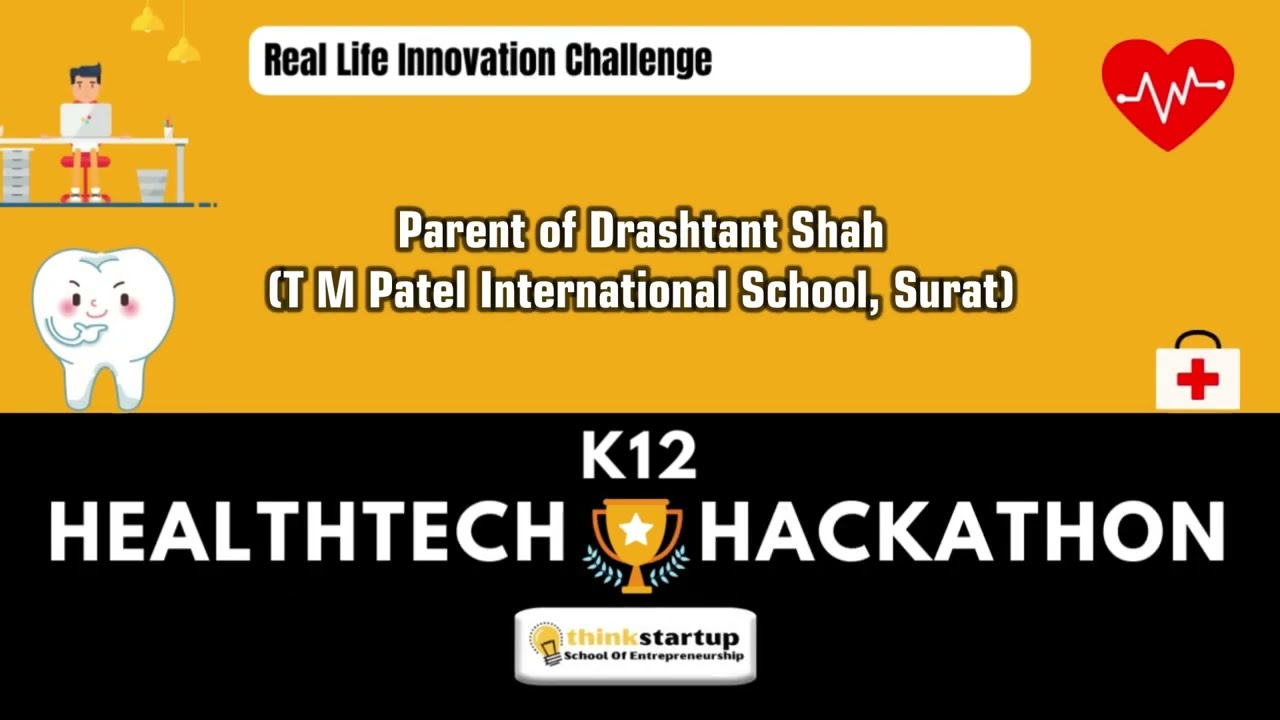The poster for the K-12 Health Tech Hackathon features a vibrant and engaging graphic design. The upper section of the image has a mustard-colored background with a white search bar at the top that reads "Real Life Innovation Challenge." Adjacent to the search bar on the left is a clipart icon of a person sitting at a desk with a laptop, creating a focused and studious atmosphere. On the upper right corner, a red heart graphic with an EKG heartbeat line symbolizes health and vitality.

Centrally located within this mustard backdrop, bold white text with a black outline states "Parent of Drashtan Shah, TM Patel International School, Surat." Below this text and to the left is an animated tooth with cheerful features, including blushed cheeks, eyebrows, legs, and hands, exuding a playful and inviting vibe. Positioned opposite the tooth on the lower right side is a white first aid kit emblazoned with a red cross, reinforcing the health theme.

The lower portion of the poster transitions to a black background, prominently displaying the event's name, "K-12 Health Tech Hackathon," in bold white text. Between the words "Health Tech" and "Hackathon," a gold trophy with a star on it signifies achievement and excellence. At the very bottom, the Think Startup School of Entrepreneurship logo is featured, grounding the event's sponsorship and focus on innovative education. Two yellow lights hanging from the ceiling illuminate the overall scene, adding warmth and focus to this bustling and dynamic illustration.